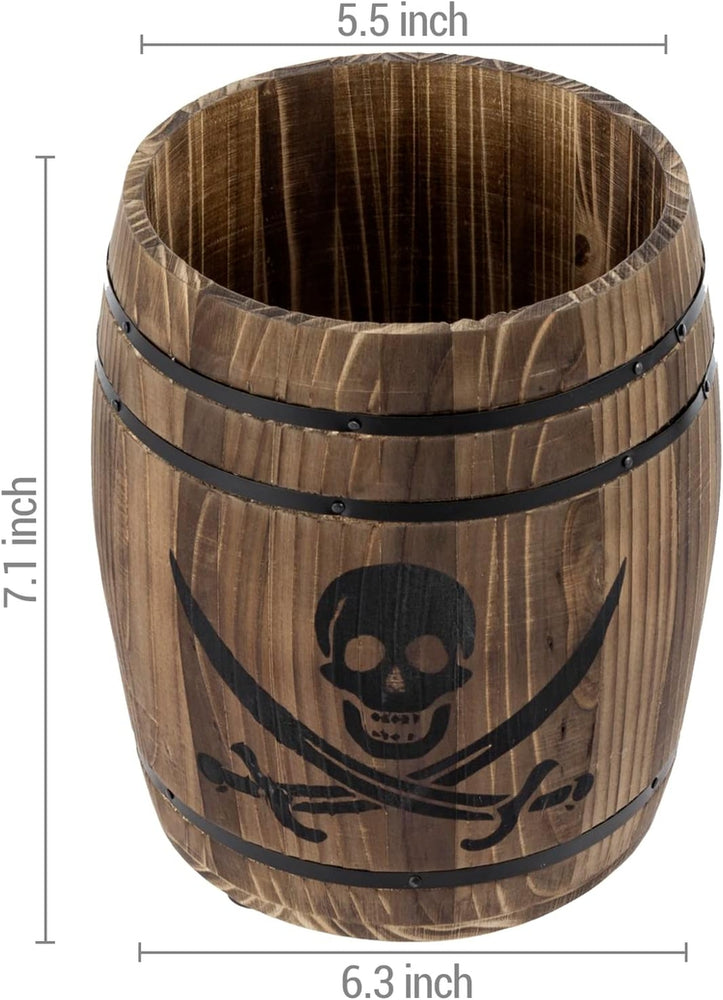This image features a small wooden barrel or a pirate's rum cask, distinguished by its rich variegated brown hues, with lighter and darker shades interspersed throughout. The barrel's exact dimensions are prominently displayed with lines and numerical measurements: 5.5 inches across the top, 7.1 inches along the side, and 6.3 inches at the base, indicating that it is a miniature rather than a full-sized barrel. It is adorned with three black metallic rings, two near the top and one at the bottom, adding to its rugged appearance. Front and center on the barrel is a black illustration of a skull with two crossed swords beneath it, reminiscent of pirate imagery, likely painted on for decoration. The skull and swords, rendered in stark black, stand out against the textured wooden surface, which varies from a drier exterior to a slightly darker and moister interior.